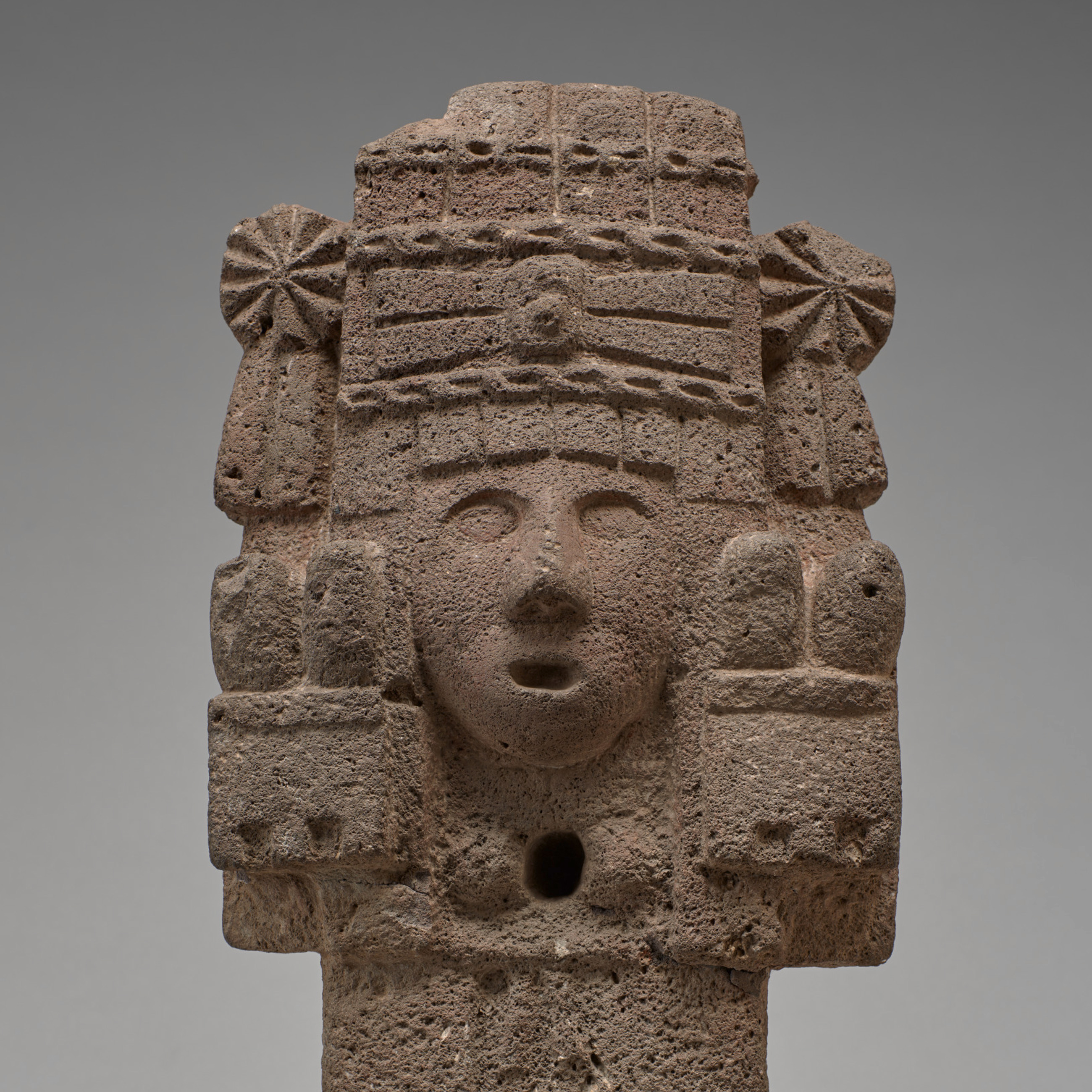The image features a detailed rock sculpture, likely made from red sandstone or cement, reminiscent of ancient civilizations such as the Inca, Aztec, or Mayan periods. The sculpture stands against a soft, medium-gray or white background. It has a rectangular base and extends outward, adorned with intricate patterns and shapes. Central to the sculpture is a youthful face with hollow eye sockets, a prominent nose, and a small oval mouth. Below the chin, there is a round hole positioned roughly where the throat would be.

Above the face, the figure wears an elaborate headdress, featuring multiple rows of chain-like designs interspersed with bars and spaces, culminating in a slightly curved top which seems to have a missing chunk. The headdress also includes square fringes and possibly floral motifs. On either side of the sculpture, there are rectangular shapes with small star-like decorations above them. The overall appearance suggests an ornate and valuable artifact that warrants preservation.